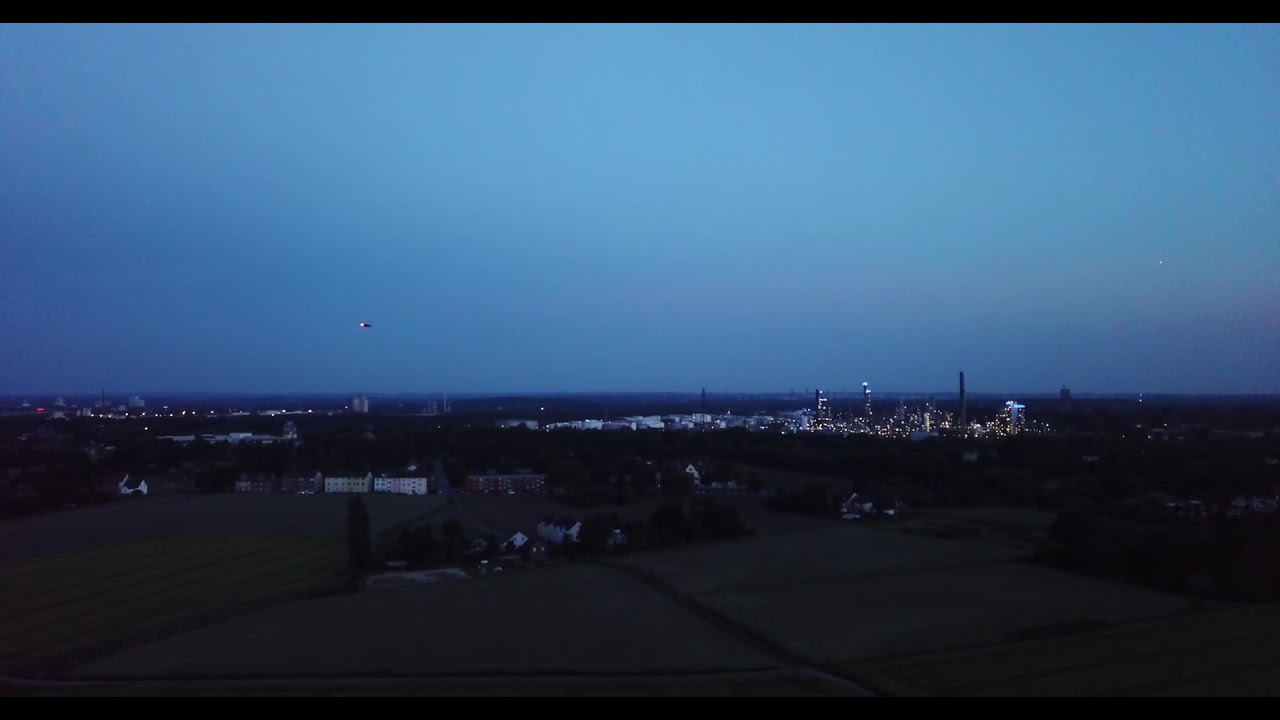This nighttime aerial photograph, captured in a wide panoramic view, presents a striking landscape scene. In the foreground, there are patches of farmland and small residential structures or farm buildings, characterized by dim lighting and a sense of peaceful isolation. As we move toward the middle of the image, the horizon line, positioned about one-third up from the bottom, separates the near-dark foreground from the distant cityscape. The city itself is a luminous collection of indistinct buildings and city lights, including three or four distinct high-rises and notable gaps possibly indicative of forested areas. A solitary tower stands on the left side, adding a unique feature to the urban sprawl. The upper portion of the image is a serene gradient of twilight blue sky, underlining the tranquility of the night. This photograph, rendered in a style of representational realism through drone photography, is inset with a black border, enhancing its landscape orientation and highlighting the subtle interplay of light and darkness.